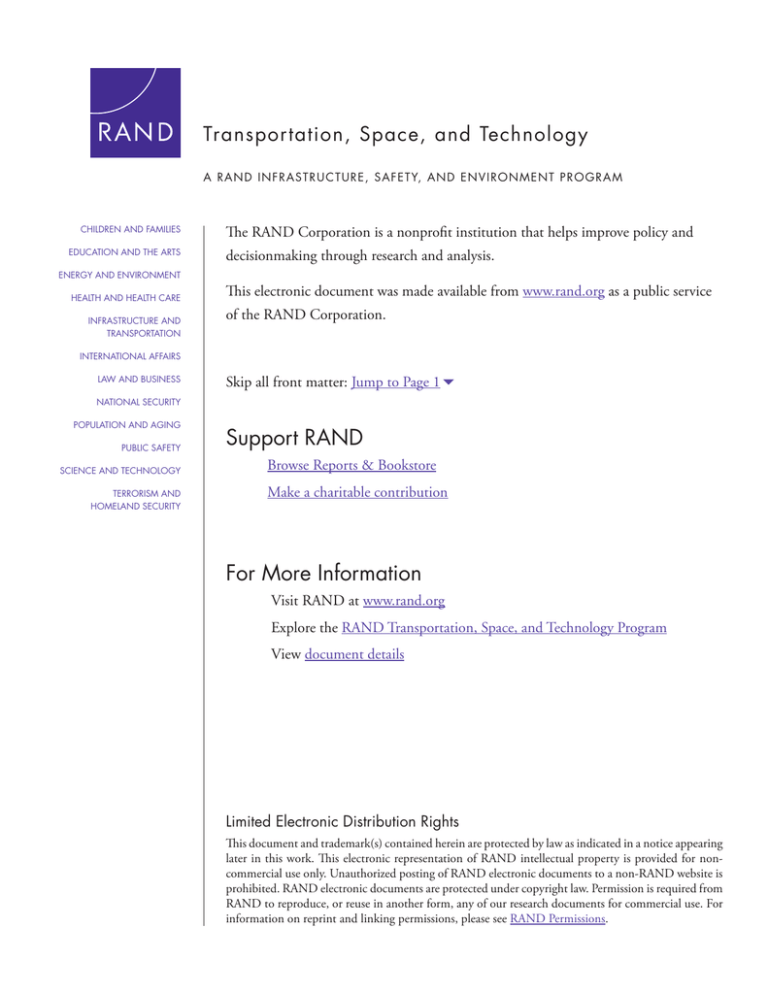This image showcases a screenshot of an internal website or webpage, set in portrait orientation against a white background with no defined borders. 

In the upper-left corner, there is a logo comprised of a red (or possibly purple) square with a white semicircle intersecting it, bearing the white text "Rand." To its right, the header reads "Transportation, Space, and Technology," with the subtitle "A Rand Infrastructure, Safety, and Environment Program" in a smaller font.

Beneath the Rand icon, a series of purple links are aligned vertically, categorized under topics such as "Children and Families," "Education and the Arts," and "Energy and Environment," among others. These links are separated from the rest of the page by a thicker vertical gray or black border.

On the right side of the border, the text explains that "Rand Corporation is a non-profit institution that helps improve policy and decision making through research and analysis." It notes that this electronic document was made available from www.rand.org as a public service of the Rand Corporation. There is an option to "Skip all front matter, jump to page 1," including a link to the first page.

Further down, under the header "Support Rand," there are two links provided. The section also encourages visitors to explore additional information and view various resources through more links. 

At the bottom of the page, there is a heading "Limited Electronic Distribution Rights," followed by detailed paragraphs outlining the document’s distribution and usage rights.